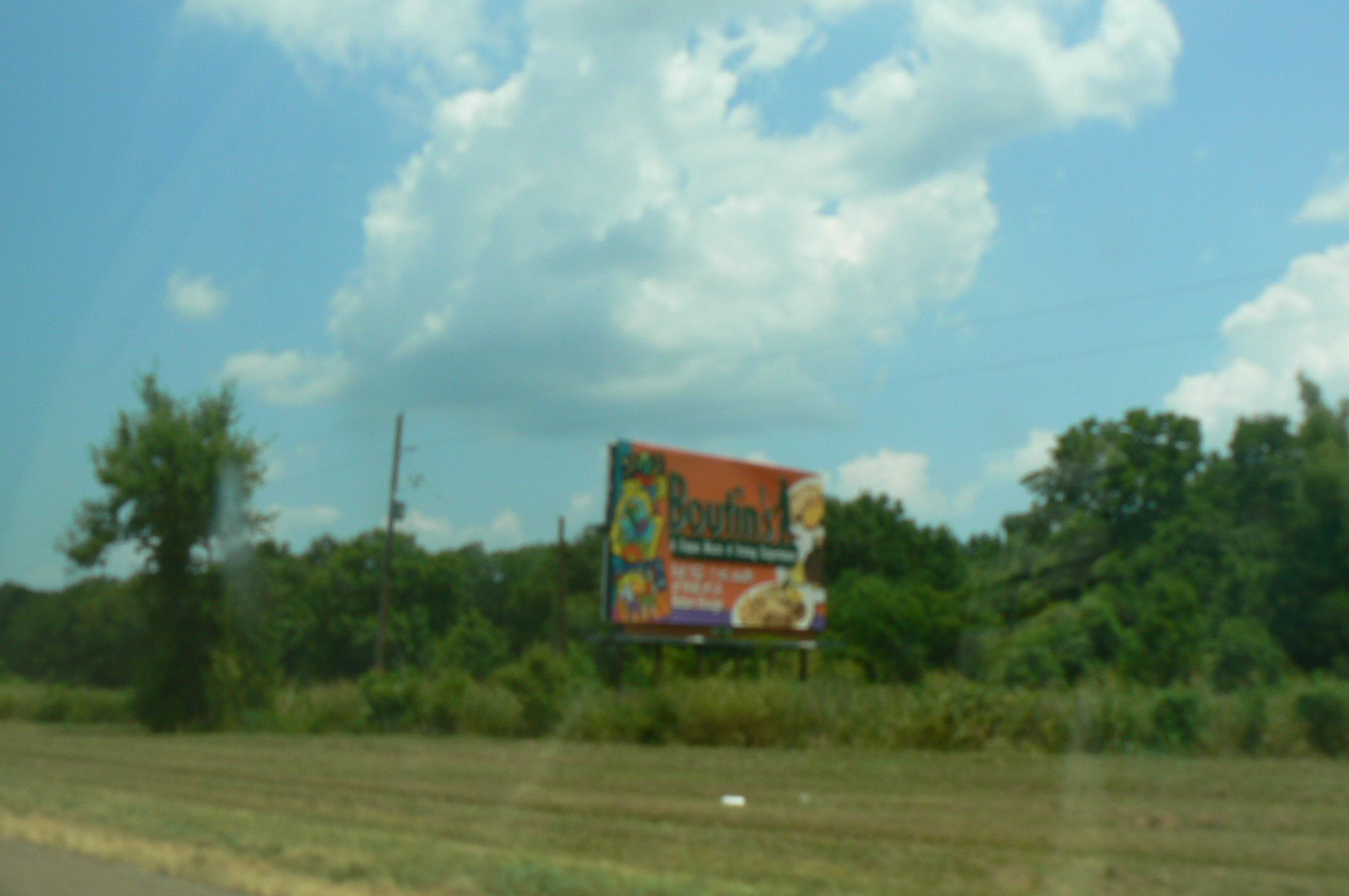This is a color photograph taken of a road sign, likely situated by the side of a road since the grey pavement with a yellow line is visible at the very lower left corner of the picture. In the foreground, some grass is present under the sign, accompanied by a small white speck that could be a reflection, indicating the possibility that the photo was taken through glass. Reflections on the grass at the bottom further suggest this possibility. 

Surrounding the sign, trees and shrubs fill the background, providing a natural setting. A blue sky with patches of grey clouds stretches behind the sign. The sign itself is partially blurred, making the text hard to decipher. The background of the sign features red and blue colors. On the left side, there is a multi-colored character, and black text is visible at the top. Towards the lower right corner, there is an image that appears to depict some kind of food item. In the middle of the sign, there's more white text, and at the very bottom of the sign, a thin blue band runs horizontally.